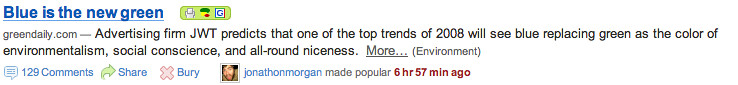This is a horizontal screenshot of a social media post from 2008 featuring a clickable blue underlined title "Blue is the New Green" on a white background. To the right, on a yellow background, are three interaction icons: a printer, a sharing icon, and a third that likely relates to Google. Following the title is text that reads: "Advertising firm JWT predicts that one of the top trends of 2008 will see blue replacing green as the color of environmentalism, social conscience, and all-around niceness." The source is noted as greendaily.com. Below this summary, there is a clickable link, indicated by the word 'environment' in parentheses, likely leading to more content. Additional details include 129 comments, share and bury buttons, and a small avatar of the user Jonathan Morgan, who made the post popular six hours and 57 minutes ago.